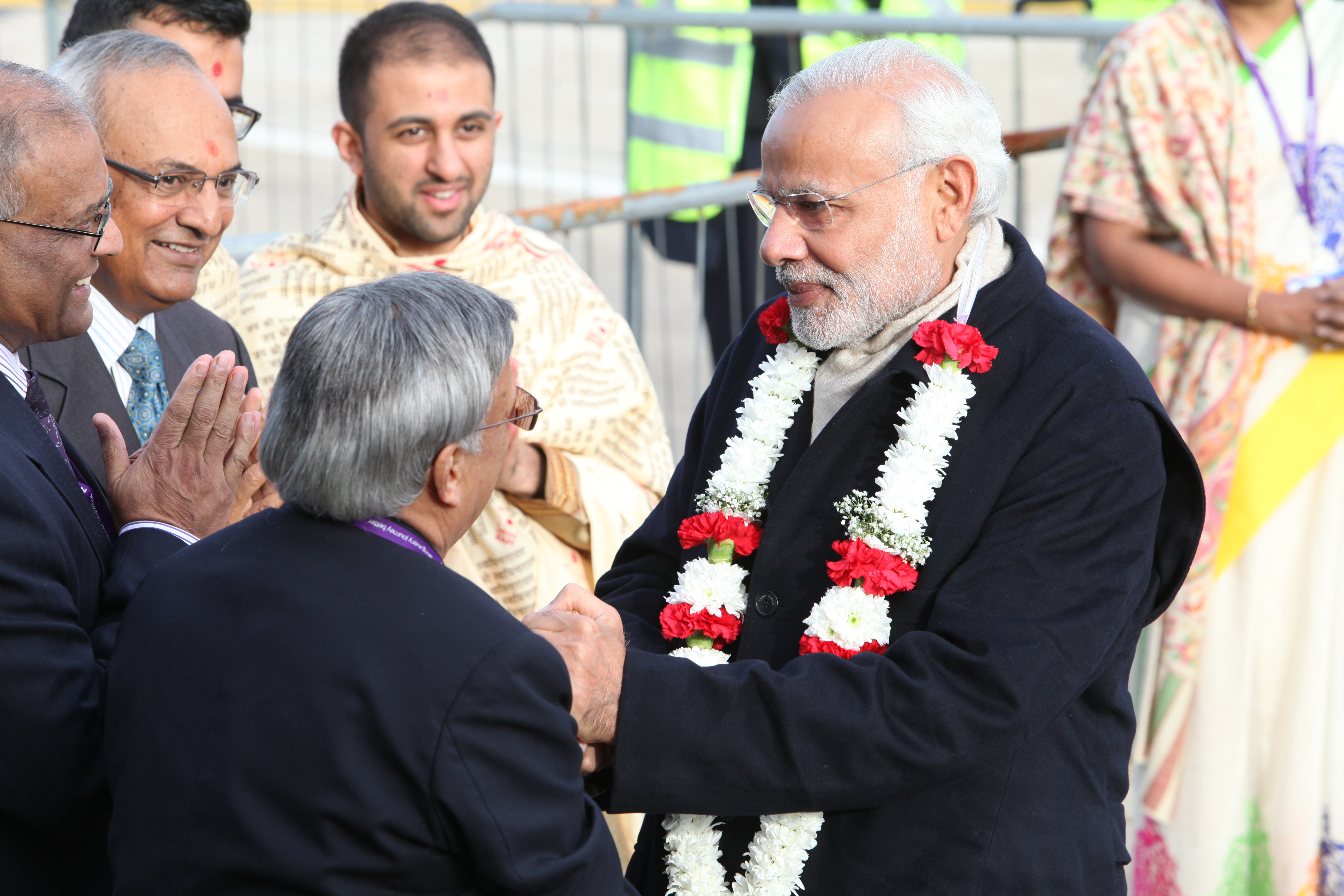The photograph depicts an outdoor scene featuring a distinguished elderly man with white hair, a white beard, glasses, a black suit jacket, and a flower lei made of red and white blooms around his neck. He stands prominently in the middle right of the image, facing a group of eclectic men. These men, who appear to be of Indian descent and dressed in either traditional garments or suits, are either looking at him or engaged in postures of respect. Two of the men in the group are attired in what resemble Buddhist monk robes. The setting suggests a multicultural gathering, possibly a political or ceremonial event. In the background to the right, a portion of a woman dressed in a brightly colored sari with floral patterns is visible. Multiple hues, including red, white, green, yellow, purple, light red, light green, and light blue, dot the scene, contributing to its vibrant atmosphere. The event appears to take place outside, with some sort of railing seen behind the group.